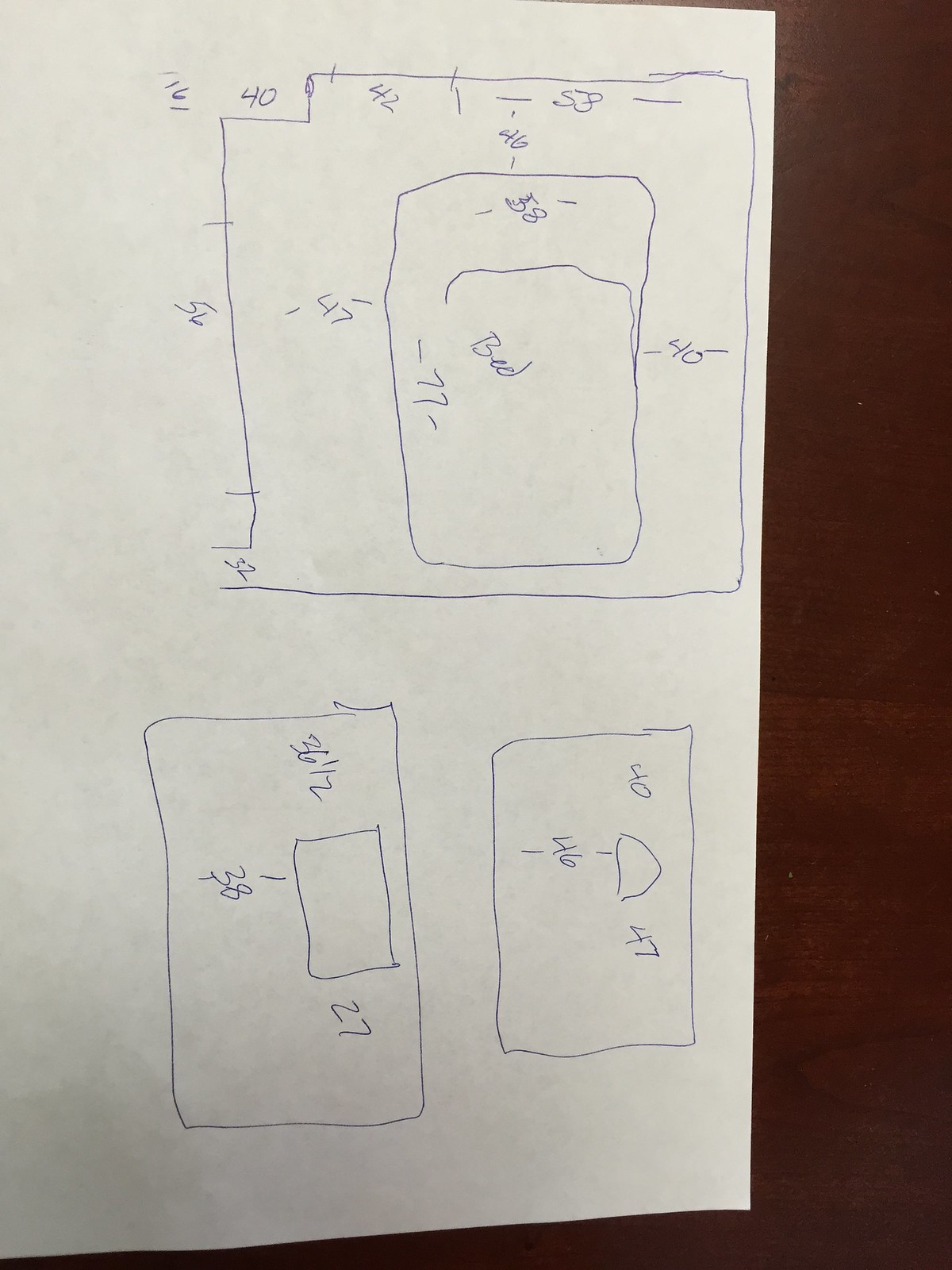The image depicts a detailed floor plan drawn on a white piece of paper, set against a brownish background, likely a wooden desk. The drawing is done in blue pen, featuring the dimensions of various rooms. The topmost section of the paper shows a large square labeled with the word "bed" in the center, indicating a bedroom layout. This square has multiple dimensions marked along its sides, with prominent measurements of 51 and 40, suggesting potential wall lengths or distances between fixtures.

Accompanying the large square are numerous additional numbers, including 77, which might correspond to specific features like closets or doorways within the room.

Below the large square are two smaller rectangular sections, each containing a box and marked dimensions. Unlike the top square, these rectangles have only three measurements each, indicating a simpler layout or smaller areas.

The intricate number of measurements and multiple sections imply that the image captures someone's detailed planning for room renovations or construction, though the precise methodology and purpose behind the numerous figures remain somewhat ambiguous.